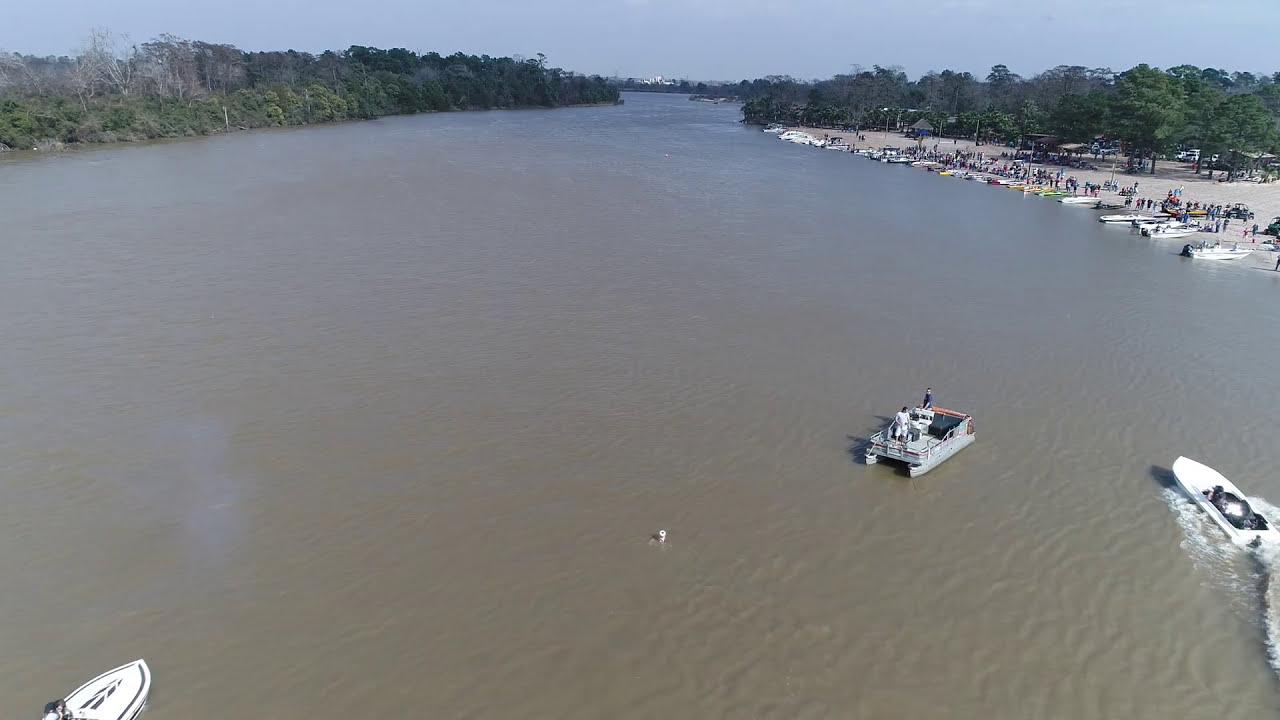This aerial drone photograph captures a vibrant outdoor scene centered around a river or lake, framed by lush green trees and flanked by mountains on the far left. The expansive water, predominantly brown, takes up much of the image and extends into the distance. On the upper right, a sandy beige beach area is bustling with tiny, almost indistinguishable people, some of whom are engaging with docked boats. In this lively beach scene, you can spot multiple boats—three of which are actively navigating the water, including one speeding boat creating a wake of white water towards the bottom right. The remaining boats are docked along the shoreline where people appear to be relaxing and watching the activity on the water. The color palette spans a spectrum of natural hues, including greens, blues, browns, grays, yellows, reds, and oranges. The background showcases a continuity of green woods on both sides of the water, with a sliver of blue sky topping the image from left to right, adding to the photograph's realistic and representational style.